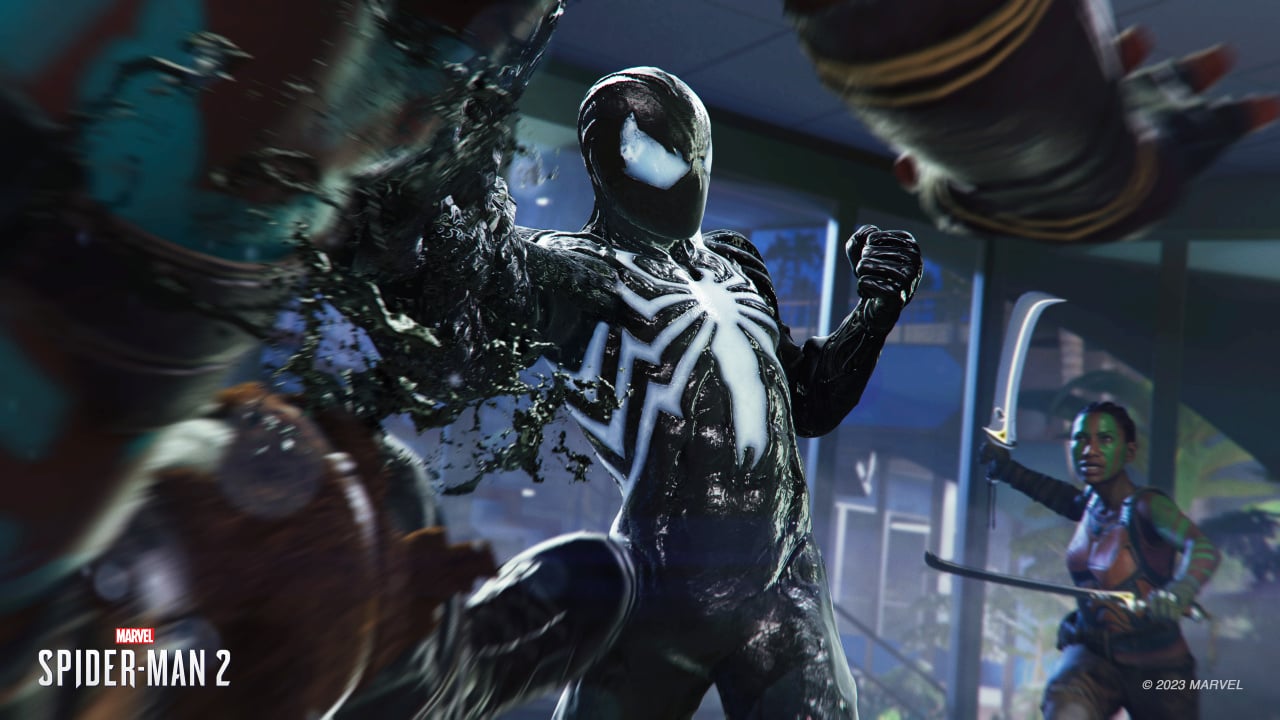In this photorealistic scene from Marvel's Spider-Man 2, Venom, depicted with a menacing black suit featuring a white spider emblem on his chest, is mid-punch, with his fist transforming into a cascading black ooze as it connects with an unseen opponent positioned off to the left. The light reflects off Venom’s rubbery texture, accentuating his intimidating presence complemented by his white eyes. The action is underlined by the Marvel’s Spider-Man 2 logo in the bottom left corner and a copyright notice in the bottom right. Positioned to the right of the scene, a fierce black woman brandishing two swords - one resembling a bayonet - looks on, either preparing to engage or already rushing towards the confrontation. The dynamic combat environment captured here suggests an intense battle unfolding, with Venom's ferocity at its core, witnessed from behind the defending individual. The inclusion of these cinematic elements gives the image a highly realistic appearance despite the computer-generated characters.